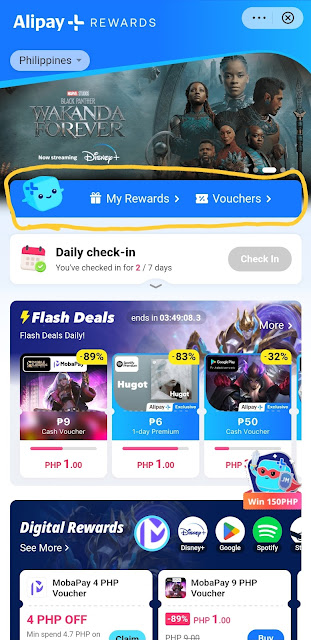Here's a cleaned-up and detailed caption for the image described:

---

A screenshot displaying the rewards section of a mobile payment app in the Philippines. At the top, an advertisement for Marvel's Black Panther: Wakanda Forever features three warriors and three priest-like figures holding staffs, standing prominently. Below the advertisement, the section is labeled "My Rewards Vouchers," accompanied by a smiling cube icon with yellow edging. The text indicates a "Daily Check-In" status, showing that the user has checked in for 2 out of 7 days. 

Further down, several flash deals are listed:
- Flash Deal: 89% off, PHP 1 voucher
- Cash Voucher: PHP 1 with 83% discount
- One-Day Premium: PHP 1 with 83% discount
- P50 Cash Voucher: 32% off, ending in 3 hours, 49 minutes, and 8 seconds

Additionally, there's an opportunity to win a PHP 150 digital reward for platforms like Disney Plus, Google, and Spotify. The user is also offered vouchers for mobile payments, including a PHP 89% off voucher and a PHP 9 HP voucher. The option to "See More" is provided at the end.

---

This caption is detailed and provides a clear and concise description of all elements featured in the screenshot.